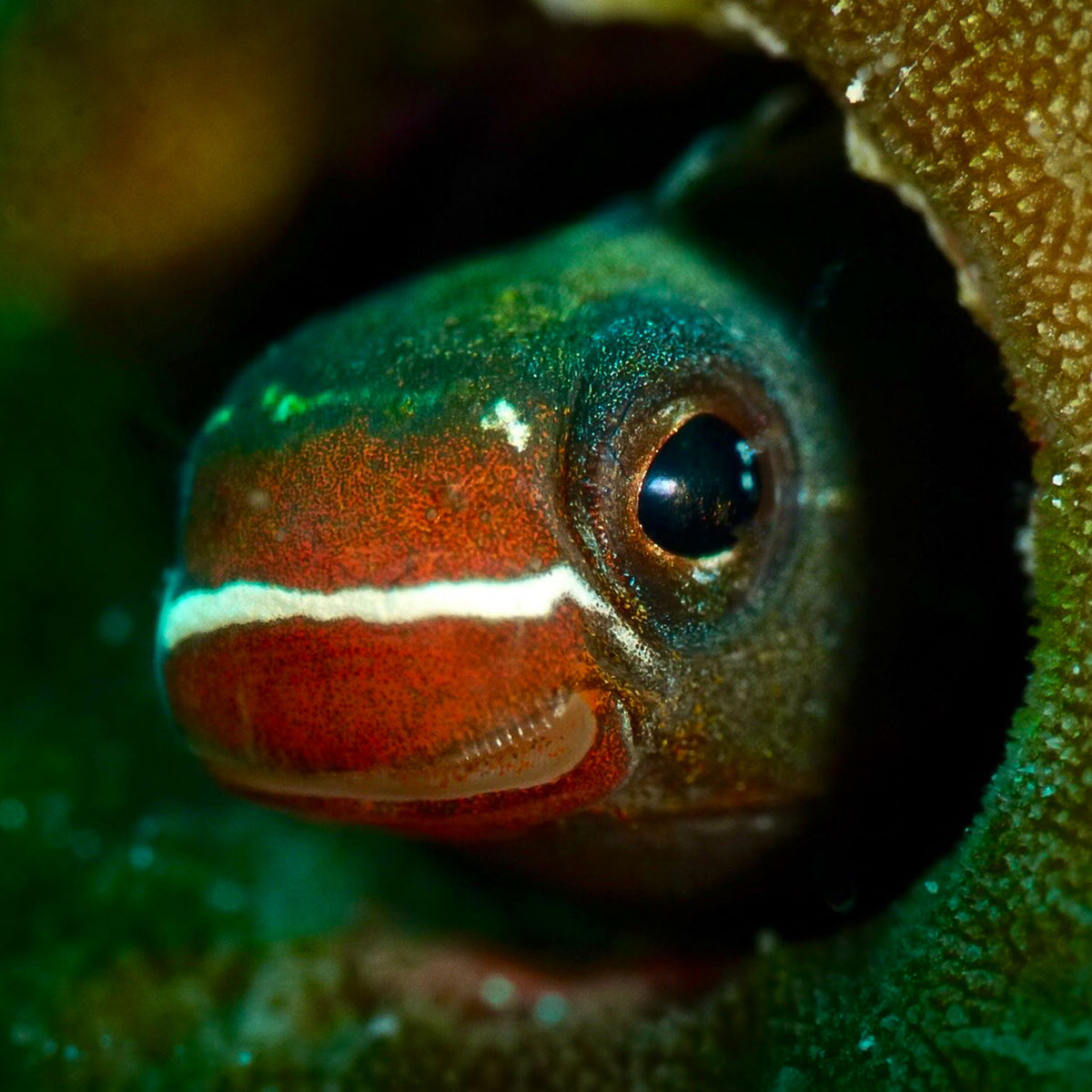This is a professional, ultra close-up photograph taken underwater of a vividly colored fish's head, likely in its natural habitat or possibly an aquarium. The fish is emerging from behind some textured, brown and green coral or rock, making the scene appear shadowy around its head. The left side of the fish's face is prominent, featuring a large, black eye encircled by shiny golden speckles. The fish displays a striking array of colors: its nose and mouth area are bright red with a horizontal white stripe, while the top of its head is emerald green with yellow and brown speckles scattered across it. The photograph captures the fish's gleaming scales and intricate details, presenting a stunning underwater portrait.